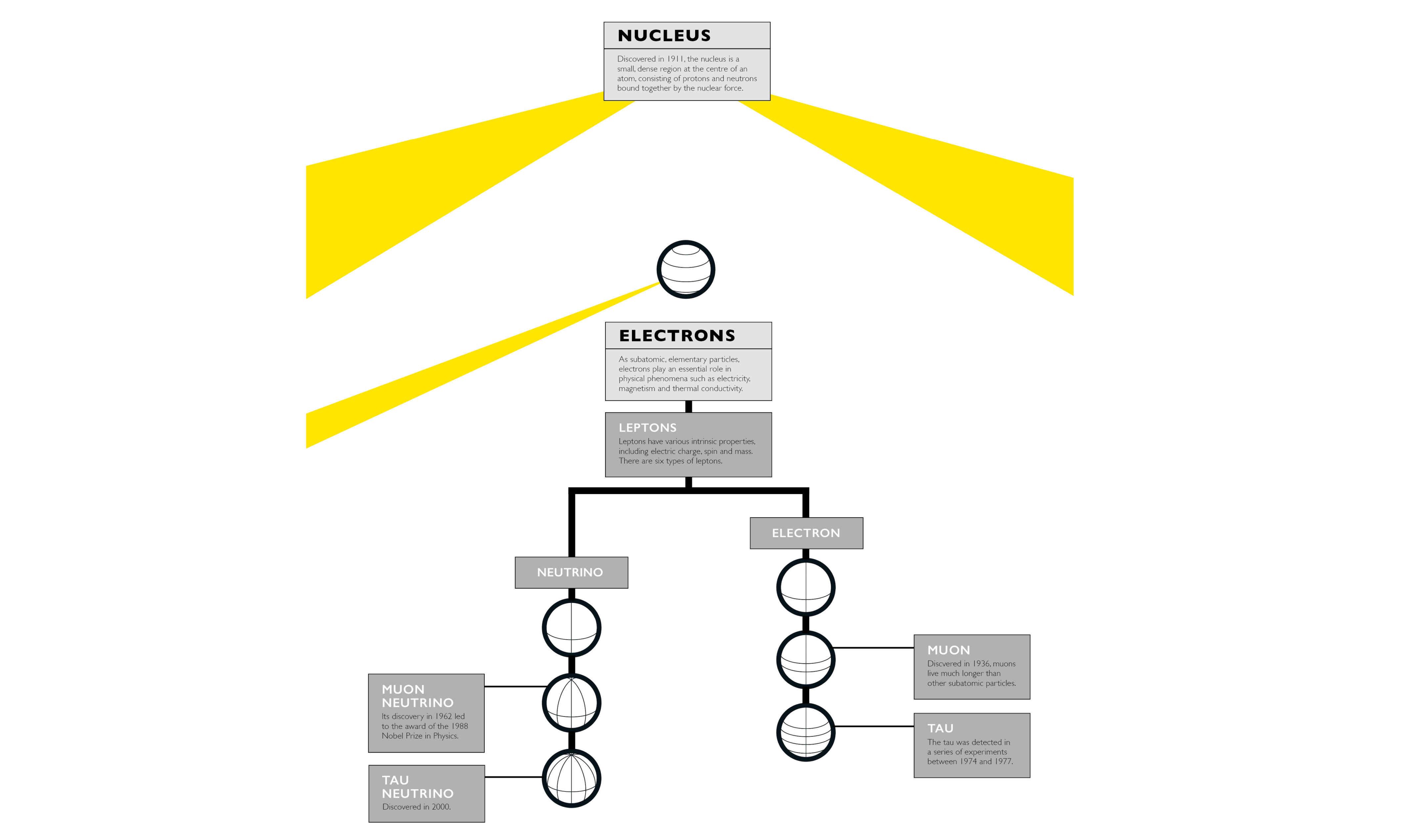The diagram illustrates the structure of an atom on a white background. At the top center, there is a light grey rectangle labeled "NUCLEUS" in bold, black, capital letters, accompanied by smaller text underneath. Extending from this rectangle are two yellow, triangular arms, one stretching to the left and the other directly downward. Below this, there is a circle with another yellow triangular arm pointing leftwards, connected to a rectangle that reads "ELECTRONS" in bold, black letters. Further below, a similar arm extends from a smaller circle, leading to labels for subatomic particles.

From the main circle, a black line branches into two paths. The left path leads to a rectangle labeled "LEPTONS," below which a black line splits into two segments. The left segment ends in a rectangle labeled "NEUTRINO," followed by three circles. From these circles, additional rectangles labeled "MUON NEUTRINO" and "TAU NEUTRINO" emerge. The right segment of the initial split leads to a rectangle labeled "ELECTRON," also followed by three circles, with further rectangles labeled "MUON" and "TAU" branching from these circles. This detailed diagram systematically breaks down the components of an atom, emphasizing the relationships between the nucleus, electrons, and various subatomic particles.